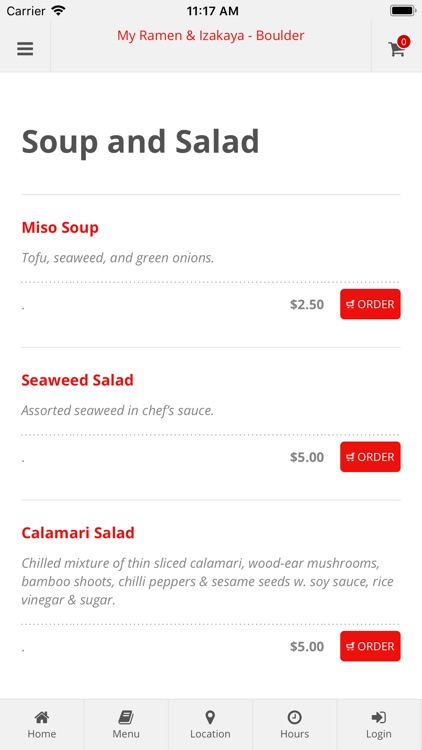**Screenshot of Mobile Application Menu**

The screenshot depicts a menu from a mobile application. At the top, a light gray header sits beneath the usual mobile icons. On the left side of the header, there is a dark gray hamburger menu icon, followed by a vertical light gray separator line. Centrally positioned, red text reads "My Ramen and Izakaya - Boulder." Adjacent to this text, after some negative space, a dark gray cart icon is present, featuring a red circle in the upper right corner, which contains a white number zero.

Below the header, the body of the page is set against a white background. At the top left of the body section, dark gray text reads "Soup and Salad." This is followed by a thin light gray separator line. The first item listed is "Miso Soup" in red text, aligned to the left. Underneath, in thin light gray italicized text, the ingredients "Tofu, seaweed, and green onions" are mentioned. This is followed by a dotted gray separator line.

To the right of the item's description, a red rectangular button with a white shopping cart icon and the white all-caps text "ORDER" is positioned. Left of this button, the price "$2.50" is displayed in dark gray numerals. A solid thin gray separator line follows this entry.

The same layout pattern repeats for the subsequent items:
1. "Seaweed Salad" - in red text, aligned left, described underneath as "Assorted seaweed in chef sauce," priced at "$5."
2. "Calamari Salad" - also in red text, detailed as "Chilled mixture of thin sliced calamari, wood ear mushrooms, bamboo shoots, chili peppers, and sesame seeds with soy sauce, rice vinegar, and sugar." Below this, "W." is mentioned, with a price of "$5."

At the bottom of the screenshot, a light gray footer contains various dark gray icons, presumably for navigation or additional options within the application.